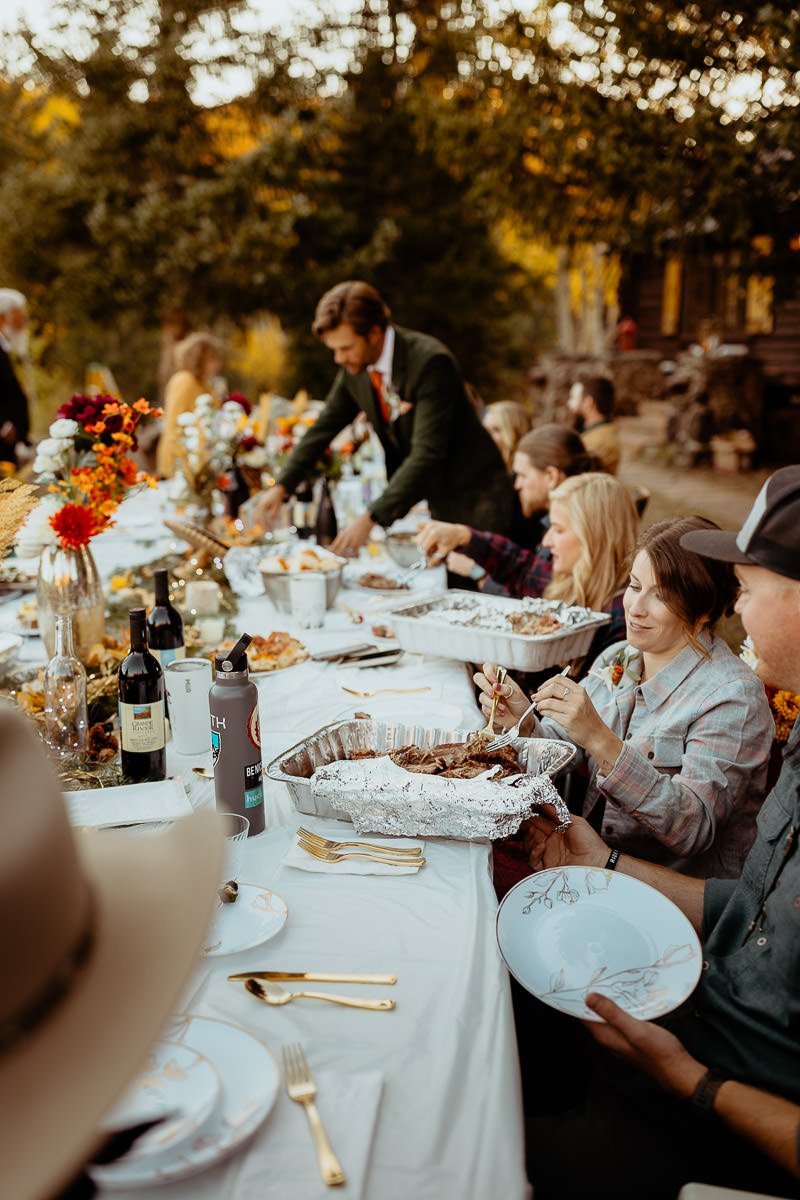This detailed and realistic photo captures an outdoor family gathering or a festive dinner party at dusk. A long rectangular table, draped with a white tablecloth, is the centerpiece of the scene, adorned with elegant gold silverware, fine china plates, and autumn flower centerpieces in gold vases. Bottles of wine are interspersed among the flowers along the length of the table, inviting guests to enjoy. A man on the left is holding a fine china plate while a woman beside him serves food from a large aluminum pan. In the background, another woman helps herself from one of several disposable metal baking dishes, while a suited man with a red tie leans over the table, adding a touch of formality to the relaxed gathering. Out of focus at the top of the photo, a tree-lined hill basked in the soft twilight glow completes the picturesque setting. The gathering is lively, with numerous guests seated and standing, engaged in conversation, and savoring a variety of foods, bread, and side dishes, creating an atmosphere rich in camaraderie and celebration.